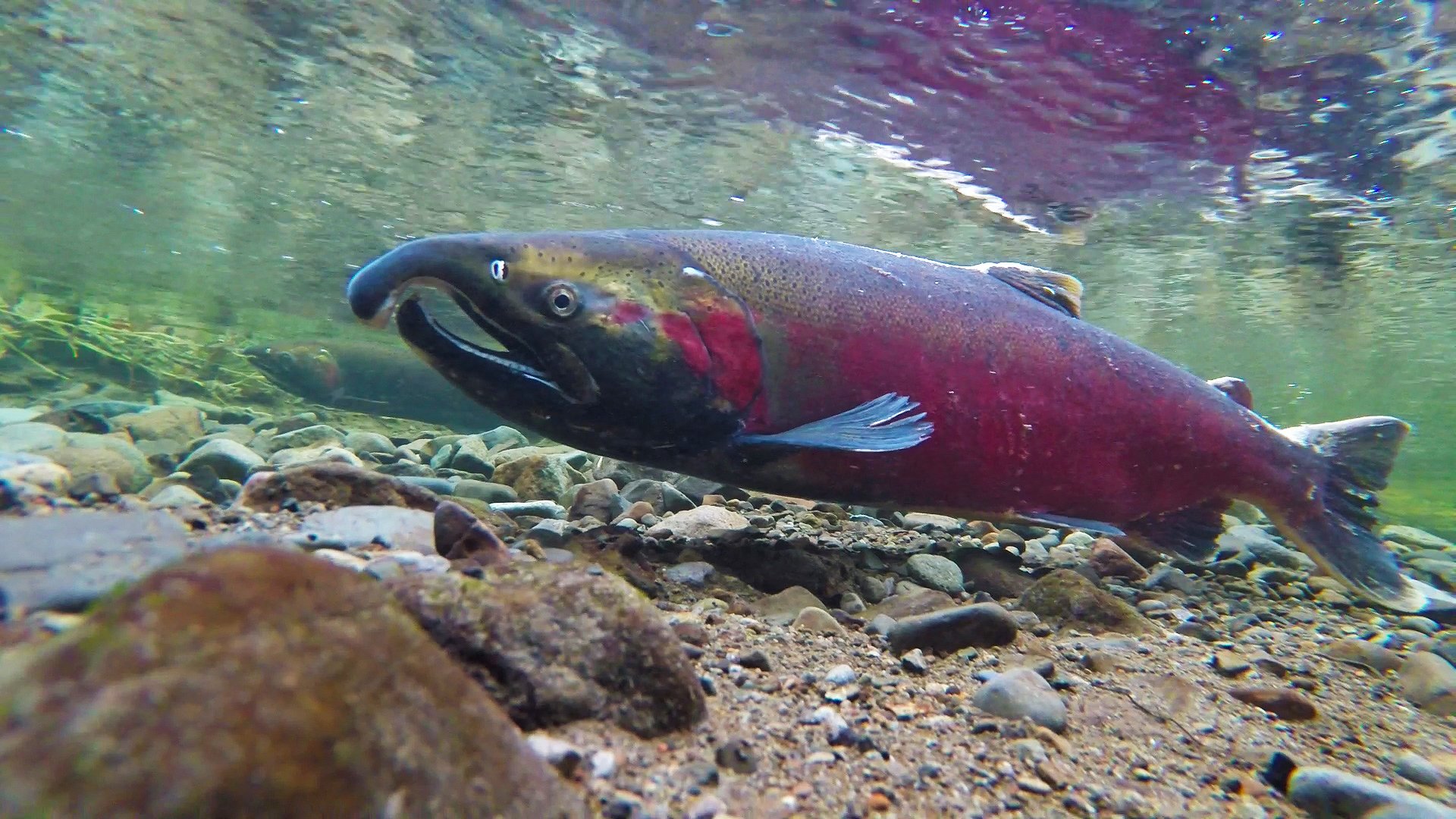This underwater photograph captures a vibrant, crimson-red salmon with a distinctive hook-shaped nose, swimming gracefully close to the rocky bed of a shallow stream, lake, or river. The clarity of the water reveals intricate details including rust-colored, gray, and small gray-brown rocks scattered on the seafloor. The water is so transparent that the surface ripples are visible, suggesting a depth of about two to three feet. The fish's body features a yellow top, black fins, and a black face with a slightly agape mouth, showing off its aquatic elegance. In the background, another similarly outlined salmon swims, contributing to the serene underwater scene. The setting’s clarity gives a glimpse of mountainous surroundings above the water, adding to the beauty and tranquility of this shallow aquatic habitat.